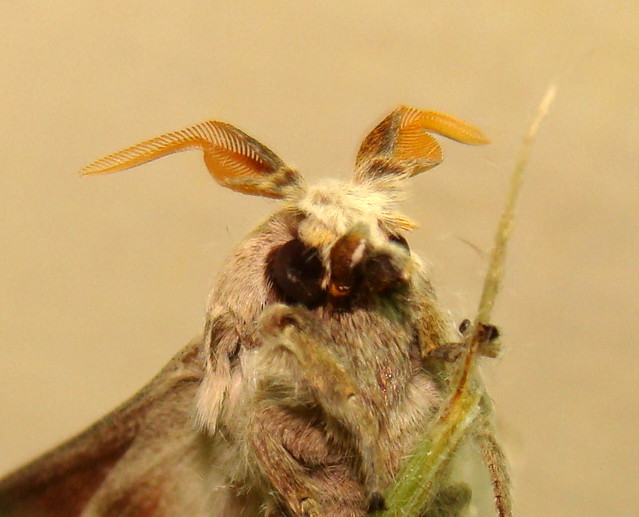In this detailed photograph set against a light brown, custard-like background, we see a close-up of a fuzzy insect perched on a slender green stem. The backdrop appears to be outdoors, as suggested by the natural setting. The insect, which resembles a moth or possibly a fly, displays a blend of light grey, white, and tan fur covering its body, with prominent brown eyes accented by dark markings around them. 

Its diminutive yet articulate hand clings to the stem, which is predominantly green with hints of brown and white near the ends. The insect's head is the focal point, facing directly toward the viewer, revealing its distinctive features: two L-shaped, ribbed orange antennas reminiscent of bunny ears protruding from the rear of its head. The body extends and slightly pushes out towards the left side of the image, with a noticeable large wing stretching from the middle to the bottom left. The wings are an intriguing mix of yellow, tan, and brown hues, adding to the detailed texture of the insect. Despite the close-up, the photograph cuts off the lower portion of the insect's body, emphasizing the intricate patterns on its upper body and head.